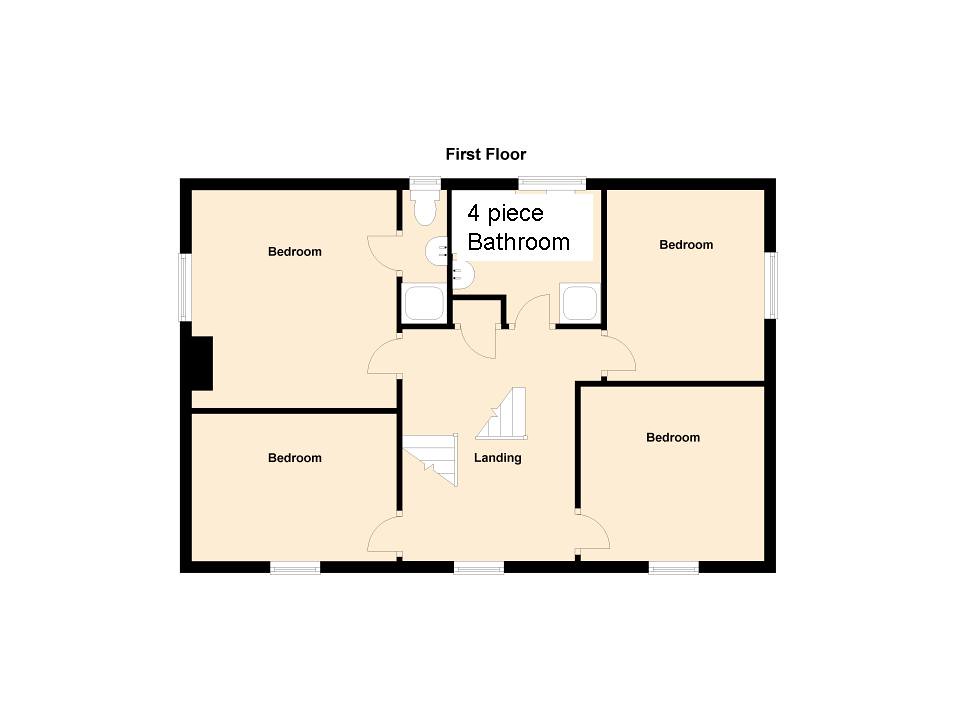This detailed floor plan of the first floor is displayed with a light pink background and dark brown outlines framing the exteriors. The layout encompasses four bedrooms: one large, one medium-sized, and two smaller ones. The floor plan also includes a four-piece bathroom. Architectural drawings of stairs are evident, with labeled "landing" areas indicating upper and lower sets of stairs. Thin black lines with slight curvature likely denote doorways, while similar lines at various points could signify either closet doors or bathroom doors. Additionally, white dashed lines around the perimeter likely indicate the presence of windows. A brown-marked area suggests the main entrance to the home.